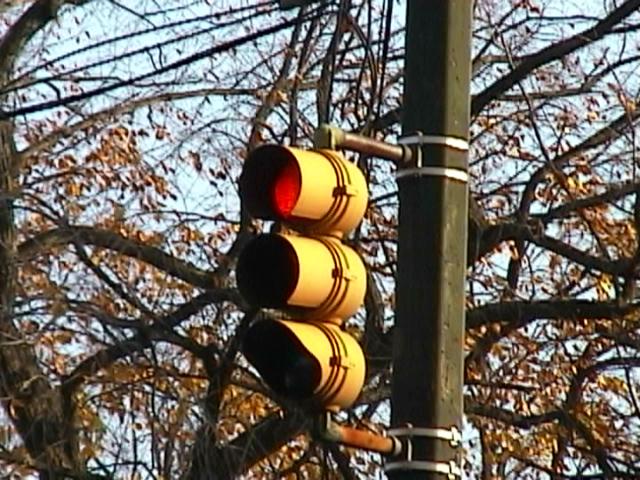In this photograph, a dark green-gray pole stands prominently in the center, supporting a vertically oriented traffic light. The traffic light, with its red signal illuminated at the top, contrasts sharply against the backdrop. Behind the pole, branches from a nearby tree are visible, adorned with sparse, yellow leaves, indicative of the autumn season. The yellow tint on the outer part of the traffic light housing suggests the influence of the surrounding ambient lighting. This serene scene captures the quiet stillness of fall, with most of the tree’s foliage already shed.